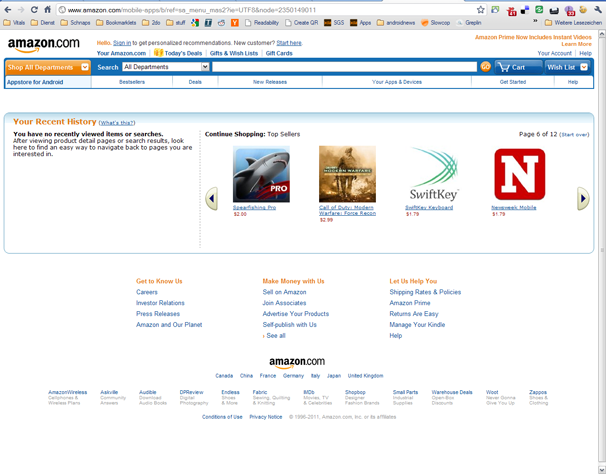The image captures the user interface of an Amazon.com webpage, as viewed in a web browser. At the top left, the iconic Amazon.com logo is prominently displayed against a white header background. Below this, the browser interface is visible, characterized by a gray top bar that houses several bookmarks and icons in the top right. Key navigational elements such as the back button and URL bar are also evident.

Directly under the Amazon logo, there is a large, rectangular orange button accompanied by a drop-down menu to its right. Adjacent to the drop-down menu is a text box positioned next to another orange button. Beneath this section, a white box bordered in blue on all sides contains the text "Your Recent History" in orange letters. Next to this phrase is a blue hyperlink labeled "What's this". Below this text, a paragraph is visible, and to its right, an image of a shark is displayed.

Additionally, the interface includes a mention of "SwiftKey" and a notable red square with a white capital 'N' in the center. Beneath this section are three columns filled with various clickable links, providing further navigational options for the user.